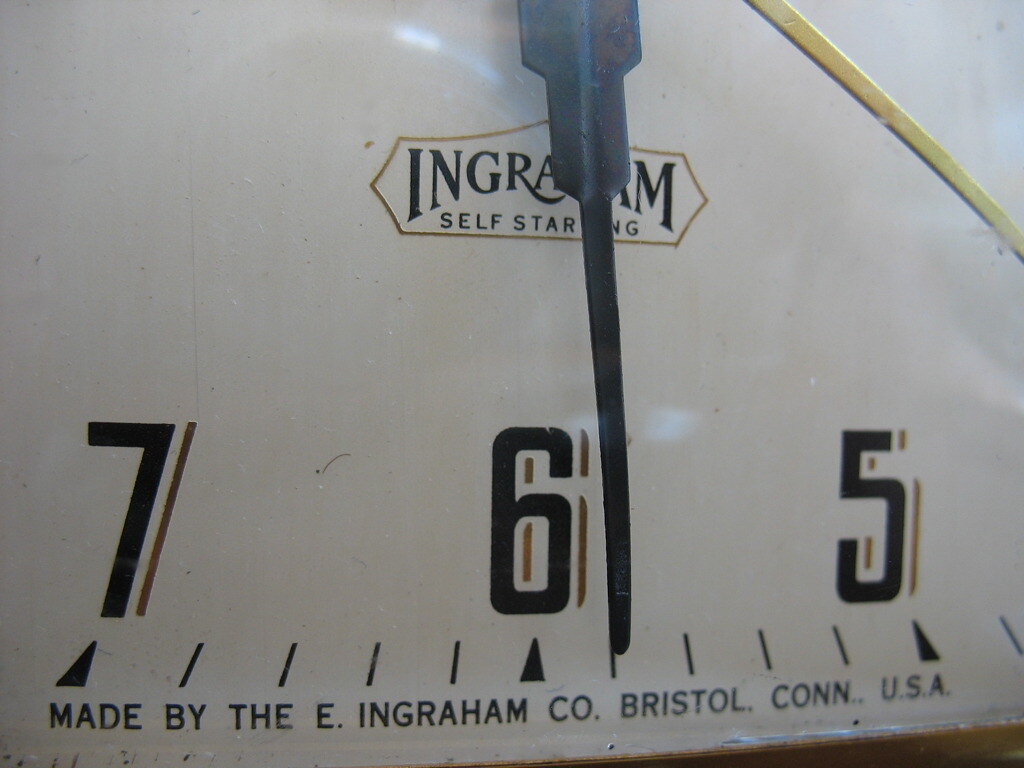The image depicts a close-up view of a partially visible clock set against a white background. The bottom portion of this object suggests it has a square frame, but most of this structure is cut off from the image. Clearly shown are the numbers '7,' '6,' and '5,' each accompanied by tick marks below them. Directly beneath these numbers, the text reads, "Made by the E. Ingraham Company, Bristol, Connecticut, USA." Visible clock hands include one potentially serving as the second or hour hand, pointing precisely at the tick mark just to the right of the number '6.' Another hand, golden in color, extends diagonally to the right, possibly indicating the second hand. The phrase "Ingraham self-starting" is partially obscured, likely by one of the clock hands. This detailed fragment provides a glimpse into the clock's intricate design and craftsmanship, though the entirety of the object remains unidentified.